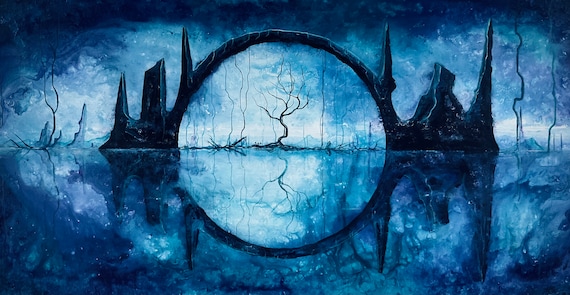This detailed and somewhat eerie artwork features a surreal landscape dominated by a striking arch made of jagged, black rock formations. The arch spans from left to right, standing over a body of water that mirrors the upper scene perfectly, forming a complete circular shape with its reflection. The scene is colored primarily in gradient hues of blue, white, and a dark swirly blue that creates a haunting atmosphere, with darker blues mixed with purples framing the edges of the artwork.

At the center of the arch, there is a barren tree, appearing wiry and leafless, adding to the desolate and creepy ambiance. The sky and reflection both give the impression of being on fire, though in cooler tones of white and blue, transitioning into a dark, swirling blue at the top. Thin branches thread through the image, enhancing the stark and spooky feeling. The overall effect is that of a dark, medieval-ish, and haunting landscape that combines elements of natural rock formations and desolate trees to evoke a sense of unsettling beauty.